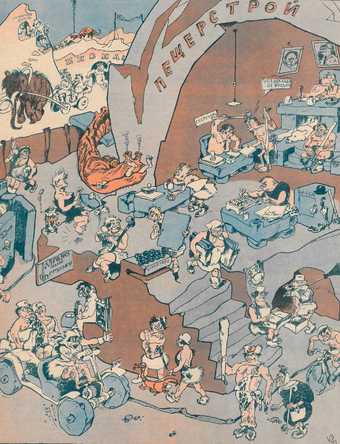This busy cartoon illustration, set in prehistoric times with a Flintstones vibe, depicts a bustling caveman-era town in muted, mostly light blue shades with hints of brown. The central focus is a large, open rock structure resembling a cavern with the cryptic inscription "N-E-W-E-P-C-T-P-E-R E-O-N" on it, possibly in a foreign language. In the upper part of the image, a woolly mammoth draws a small cart carrying two people. Below, various cavemen, clad in rough, animal-skin loincloths, engage in numerous activities, utilizing stone-made furniture. In a bustling scene, a man angrily gestures from behind a stone desk in a makeshift office, while another person reclines on a stone couch. To the left, a dinosaur extends its neck from behind the building, ominously holding a partially eaten figure in its mouth. Additionally, a crude vehicle with stone wheels, peddled by a front driver, appears alongside another primitive car with ancient tires. The image teems with energy and detail, capturing a lively, albeit chaotic, snapshot of ancient, inventive life.